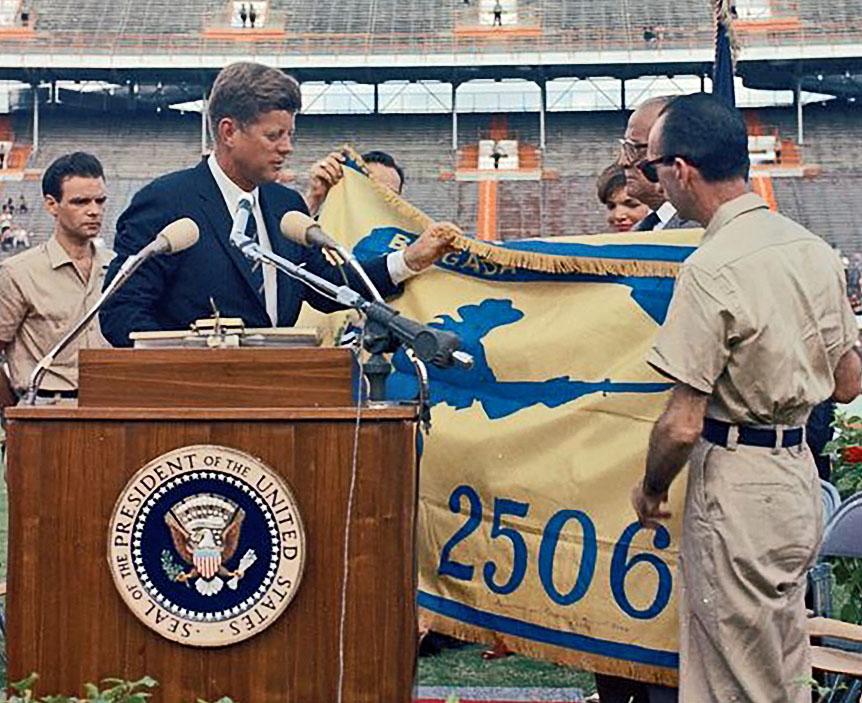In this vintage color photograph, former US President John F. Kennedy is captured standing to the left side, behind a dark wooden podium adorned with multiple microphones. The podium bears the official "Seal of the President of the United States," featuring a bald eagle holding an olive branch. Dressed in full business attire, Kennedy is intently gazing to his left towards a prominent blue and gold banner displaying the numbers "2506" and a cowboy-like silhouette brandishing a bayonet. 

This significant flag is being held by several men in khaki uniforms, suggesting possibly a military background, who are all gathered around Kennedy, presenting the flag for his review and approval. In the background, a large stadium filled with bleachers can be discerned, with several figures visible at different levels, indicating a public or secure event meant to protect the President. Among the crowd, Jackie Kennedy can be spotted, enhancing the historic gravitas of the scene. The overall atmosphere evokes a sense of solemnity and ceremonious respect, fitting for an event from the early 1960s.